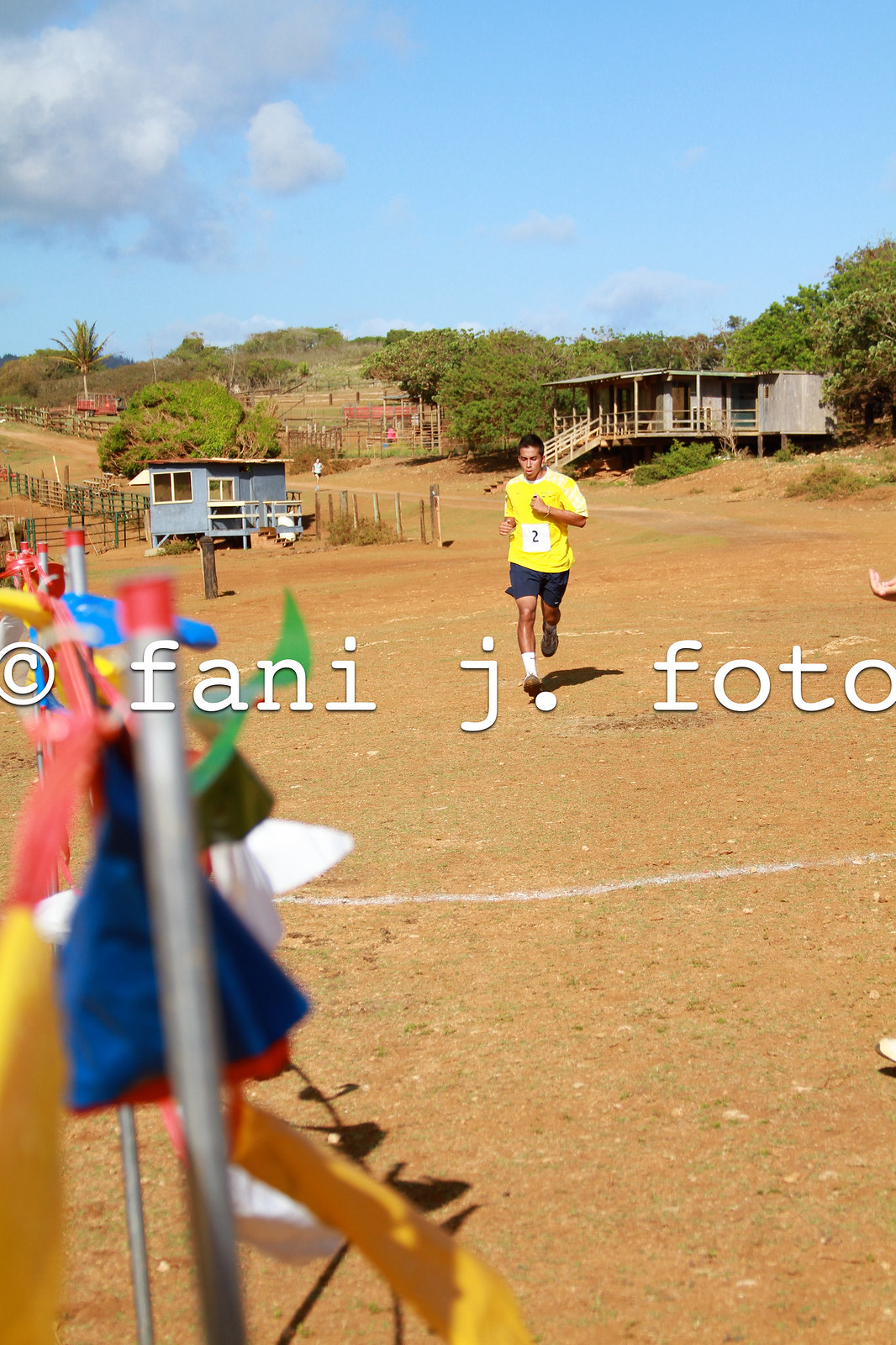In a vibrant outdoor setting, the photograph captures a man with brown skin running energetically, adorned in a yellow and white shirt, blue shorts, white socks, and light brown shoes. Prominently displayed on his front is the number 2. The scene unfolds on a dirt road lined with what appears to be the finish line etched in white in the foreground. Surrounding him is a picturesque landscape featuring a mix of green trees, possibly a palm tree, and wide open spaces, indicative of a ranch-like area with scattered fence posts and a couple of homes. In the backdrop, various colorful flags flutter near the homes. Despite the ambiguities of his exact activity—be it a marathon or a soccer match—the scene is branded with the text "Fanny J. Photo," adding an artistic touch to the lively moment under a mostly clear sky with a few clouds.